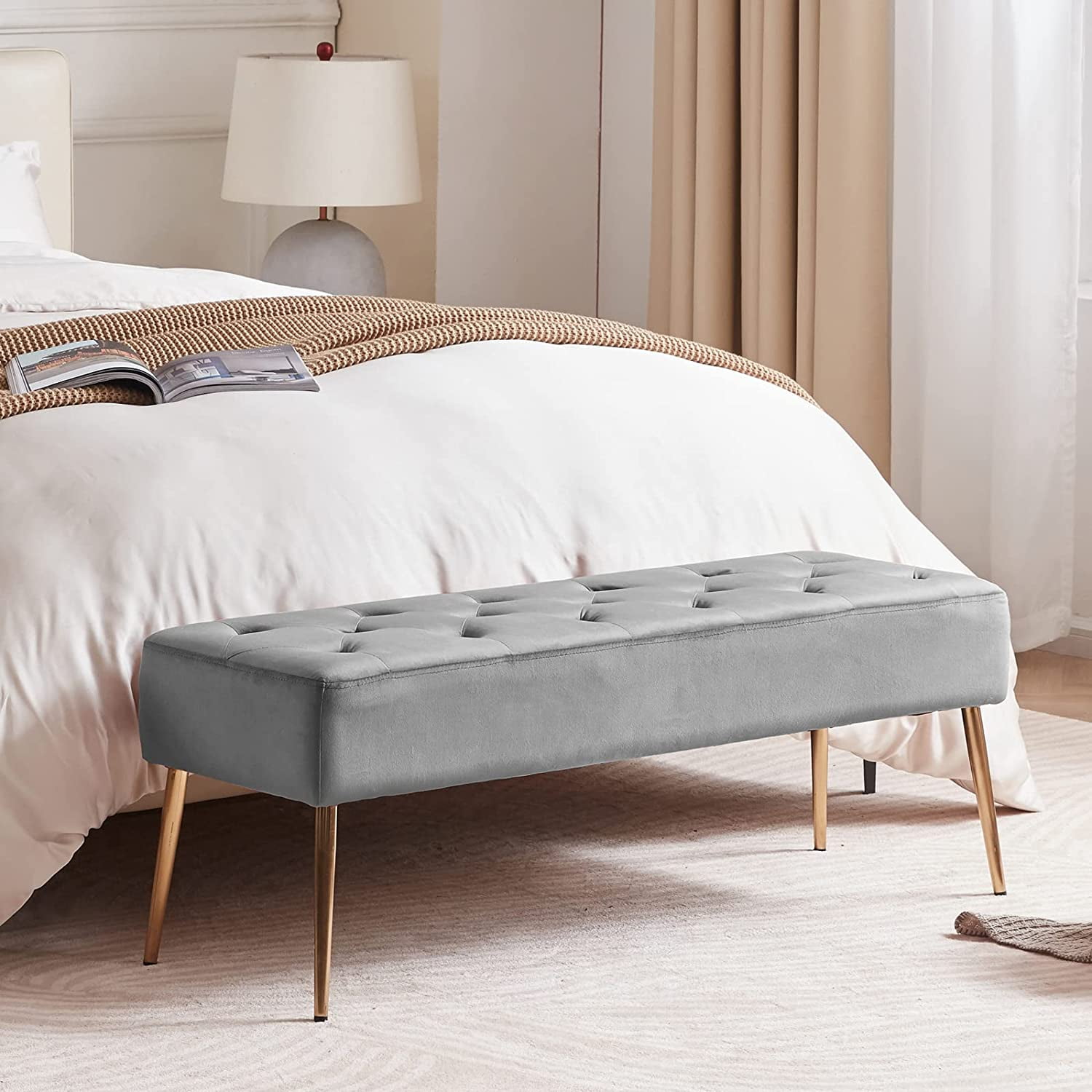The photograph depicts a cozy bedroom characterized by a soft, neutral color palette dominated by beige and cream tones. The background features a beige-colored wall with a window covered by long, white drapes and cream-colored curtains. Alongside the window sits a bed with a cream-colored headboard. The bed is dressed in a thick cream bedspread, complemented by a brown woven throw laid across the bottom, on which an open magazine rests.

At the foot of the bed, there is a plush, velvety gray stool with slender, gold legs capped with black tips. The floor, in front of the bed, is covered with a light pink carpet, adding a subtle touch of color to the room. To the right of the bed stands a bedside lamp, featuring a gray base and a cream-colored lampshade. The room exudes a serene and elegant atmosphere, perfect for relaxation.